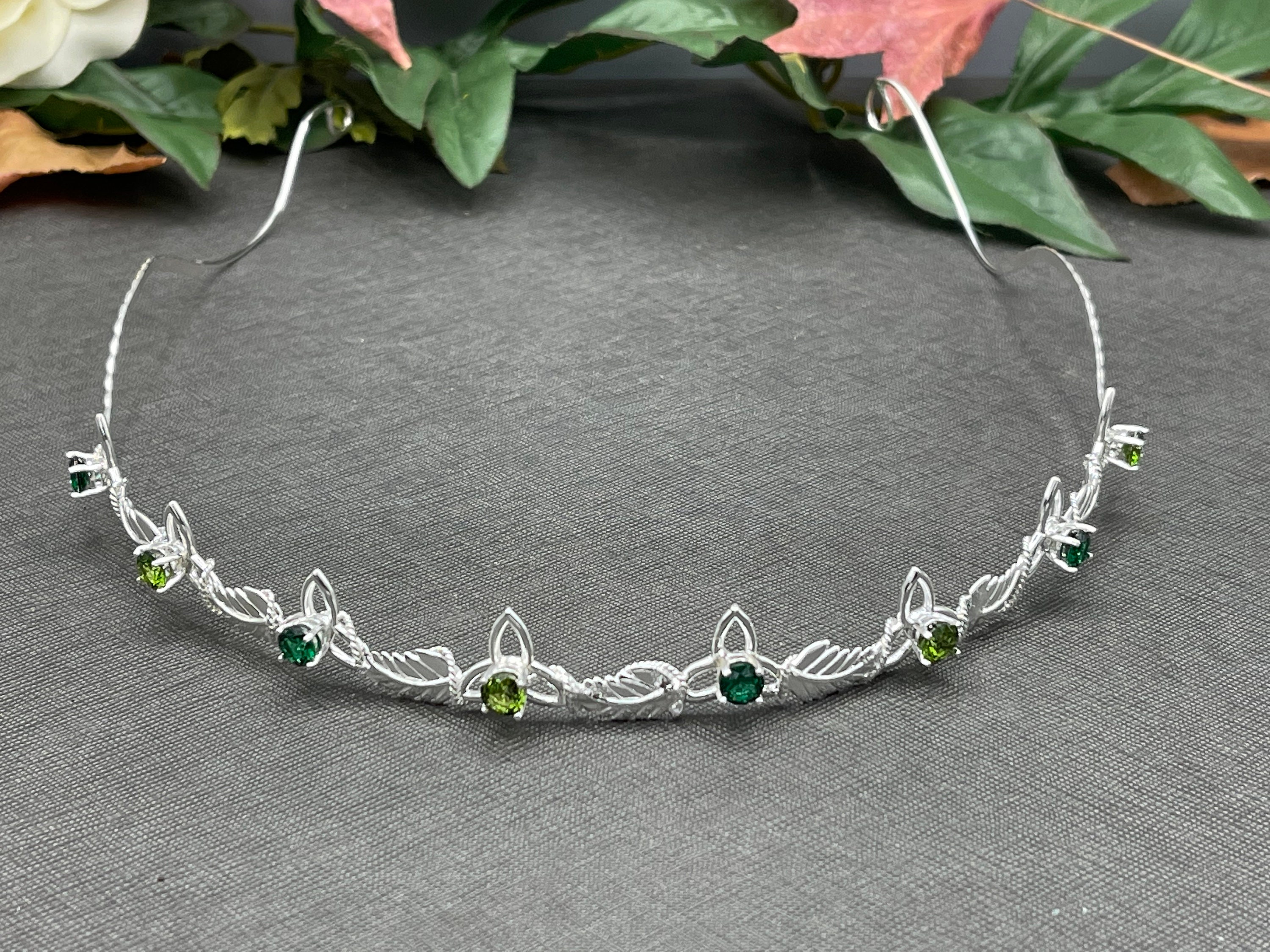The image features a delicate, thin, wiry silver tiara prominently placed on a gray fabric surface. The tiara is intricately designed with elegant curls at the back and rises to meet the front where it displays a series of small flower-like designs adorned with alternating dark and light green gemstones, each set about an inch apart. The gems are carefully arranged in an alternating pattern starting with dark green, followed by light green, and continue this sequence across the length of the tiara, totaling eight stones. The background showcases lush, thick green leaves that span the entire top part of the image, adding a natural, vibrant contrast to the scene. Additionally, there is a noticeable red flower on the upper left corner, and a white flower on the upper right corner. Near the center of the background, pink petals or a pink flower can be identified, contributing to the rich botanical backdrop.